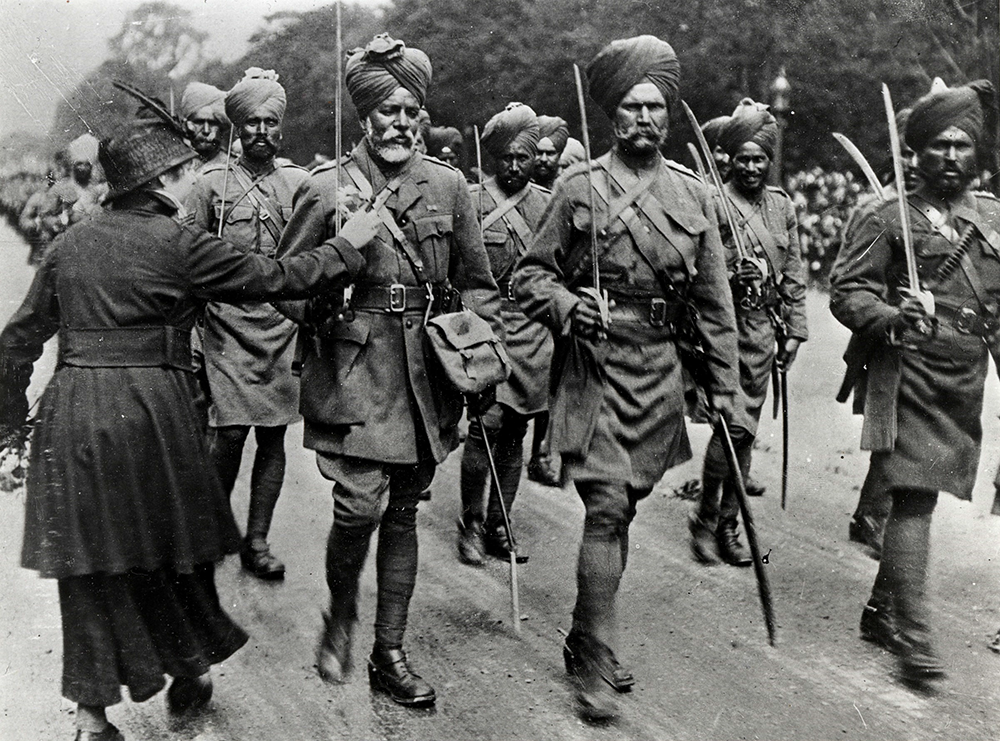This black-and-white historical photograph depicts soldiers marching in a disciplined formation down a dirt road, set against a backdrop of a lush tree line. The soldiers are walking in lines of three, clad in military uniforms featuring long coats or short skirt-like suits with crossbody artillery belts. Each soldier wears a turban and boots, and they carry swords upright in their right hands. Their somber expressions are accentuated by their prominent facial hair, including handlebar mustaches and beards. On the left side of the photo, a woman in a dark dress, long jacket, and hat is reaching out to touch the chest of the soldier closest to her. This soldier stands out with his white mustache and beard, and his coat that descends to just above his knees. The formation continues into the background, with additional soldiers visible in the distance, maintaining the disciplined structure of the march.